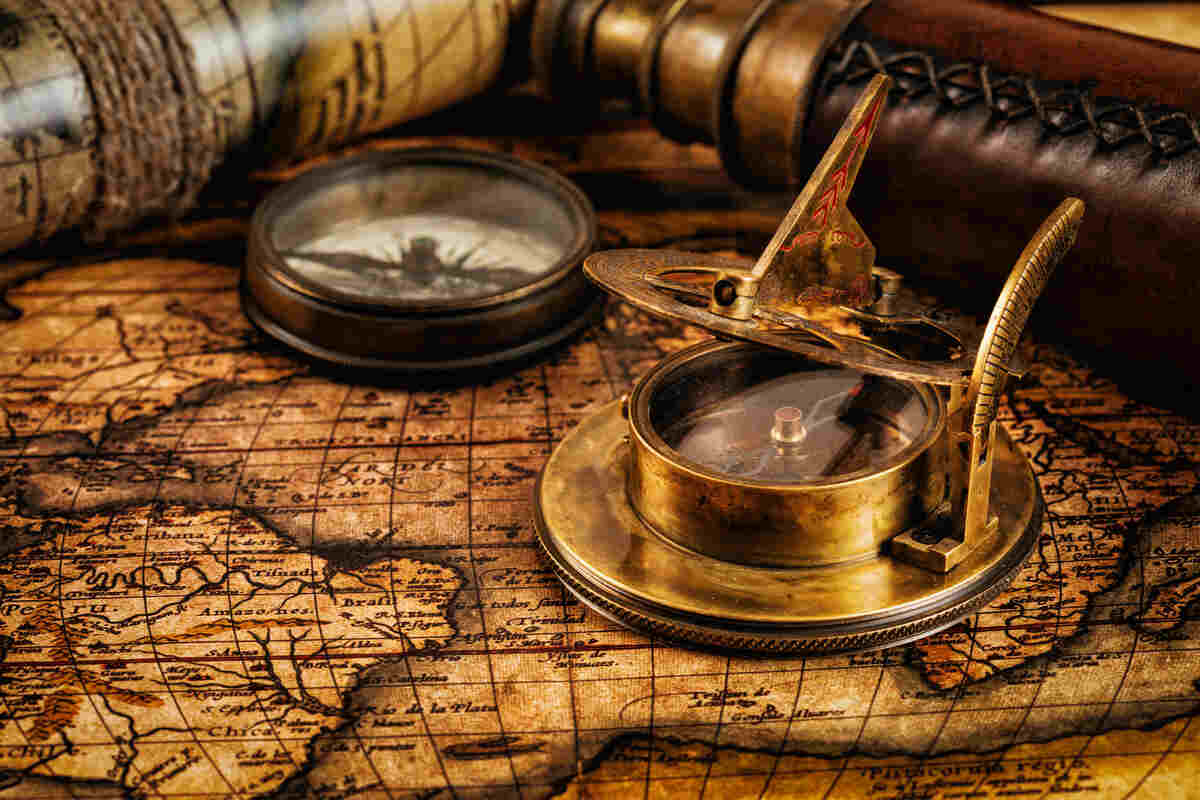This highly detailed, photographic image appears to be digitally enhanced, likely with Photoshop, to boost color saturation and contrast. It features an old world map laying flat as the background. On this map, two main objects stand out: a traditional metal compass sitting prominently at the bottom right, and another slightly different, golden compass positioned nearby, both with dual pointers. The scene is rich in hues of bronze and burnt sienna, highlighted by studio lighting. Additionally, a wooden instrument with a glass cover and a leather item are visible, though slightly out of focus, adding texture and depth to the composition.